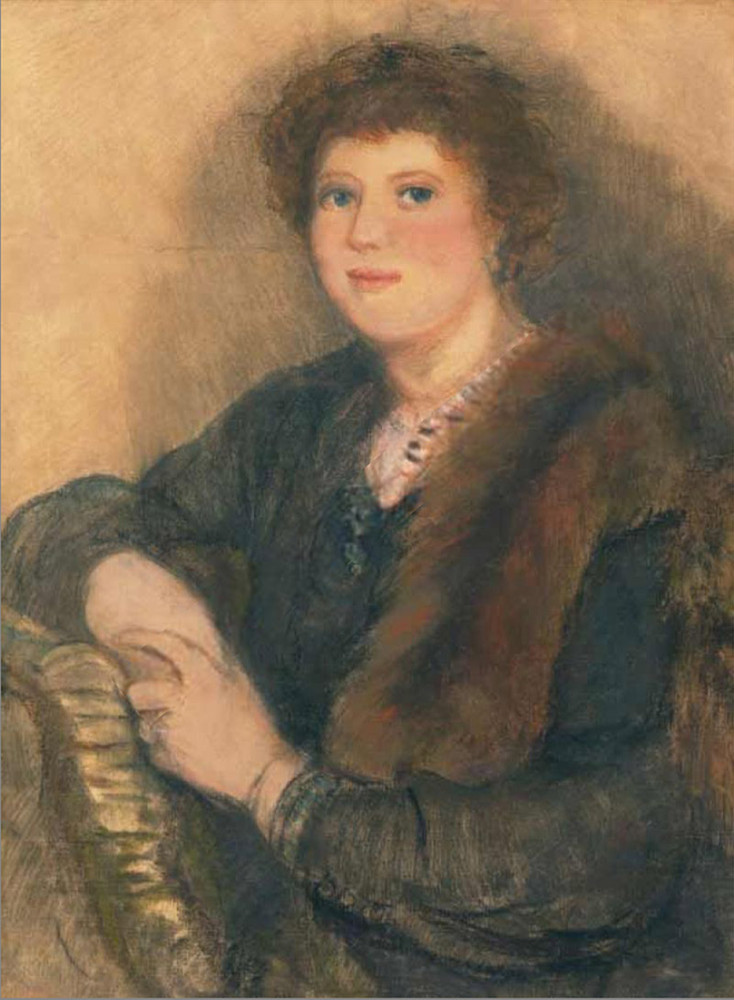This painting depicts a woman, approximately 38 years old, seated in a detailed and graceful pose. She wears a long-sleeved dress in a blend of dark gray and brown hues. Her right arm rests elegantly against the back of what appears to be a chair or perhaps a couch or chaise, while her left hand, adorned with a ring on her ring finger, lightly touches her right hand in front of her. Draped over her left shoulder is a distinctive fox fur shawl.

The woman has short, wavy, and curly brown hair, framing her symmetrical, round face with red rosy cheeks. Her expression is pleasant as she gazes towards the viewer with her large, striking blue eyes. A necklace, resembling pearls with some of the beads being larger or darker, adds a touch of elegance to her attire.

The background of the painting features a dark charcoal brown, with gradient shading that accentuates the figure of the woman. Despite the shadowy tones of the artwork, there is a certain warmth and vibrancy to the overall image, capturing the subtle details of the woman's attire and features beautifully.